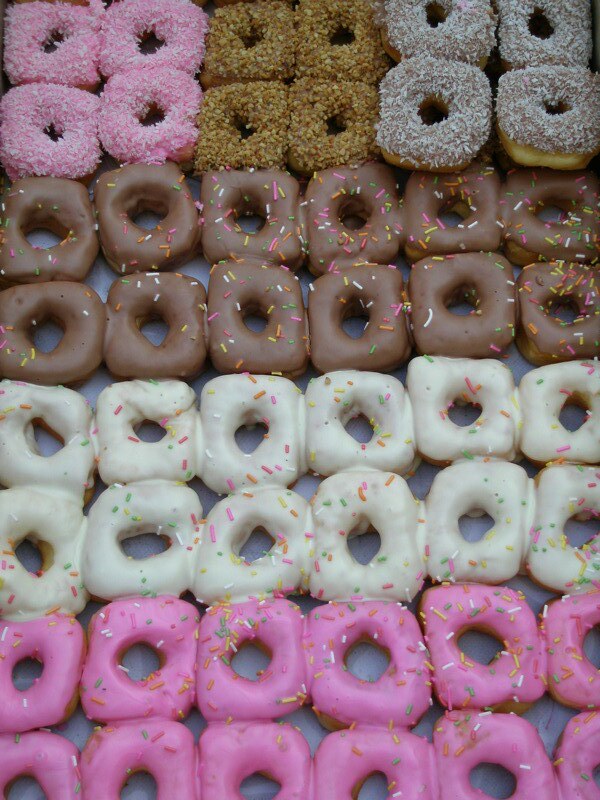This is a top-down photograph depicting a meticulously arranged display of 48 doughnuts in a vertical, rectangular grid. The doughnuts are slightly square-shaped and all closely packed together on what appears to be a sheet of white wax paper. There are eight rows and six columns, perfectly filling the entire frame with no background visible. Starting from the top, the first row features an assortment of crumb-style doughnuts: four on the left have pink frosting with white sprinkles, four in the middle are coated in brown crumbs (possibly peanuts), and four on the right have white crumbs. The next two rows below consist of 12 chocolate-covered doughnuts adorned with colorful sprinkles, followed by two rows of 12 doughnuts with white frosting and colorful sprinkles. The final two rows at the bottom showcase 12 doughnuts with pink frosting and colorful sprinkles. The overall aesthetic is vibrant and visually pleasing, with the colorful sprinkles adding a lively touch to the neatly organized doughnuts.